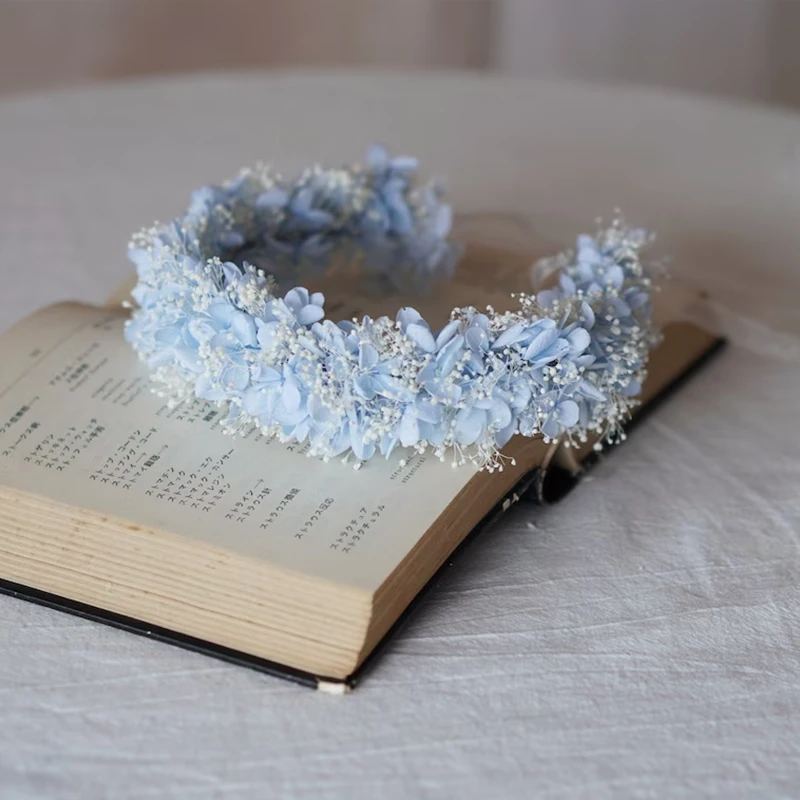This image features an open, worn book with a black hardback cover and tan-white pages, placed on a textured white tablecloth draped over a round table or stand. The book's text is not in English; it might be in Korean or Japanese, though it's not clearly identifiable. The left-hand page is visible, while the right-hand page is obscured by a decorative headband resting on top. The headband, shaped like a horseshoe or three-quarters circle, is adorned with blue and white flower designs. The background of the image is blurred, highlighting the book and headband as the main subjects.